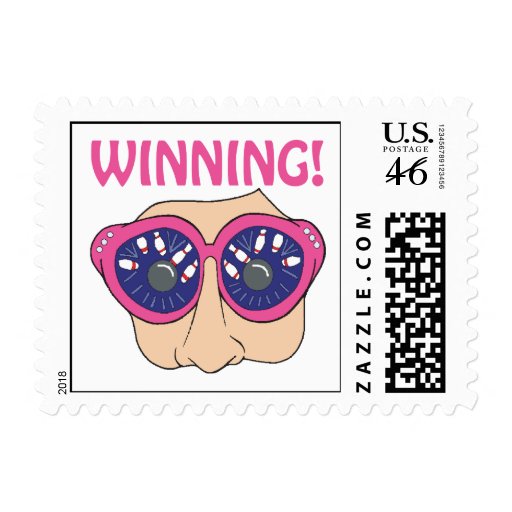This image features a postage stamp with a detailed, cartoon-style drawing placed against a solid white background. The central figure is a human face with fair skin, adorned with a pair of pink-framed glasses. Intriguingly, the reflection in the glasses showcases a scene of a bowling ball striking five bowling pins, mimicking the figure's eyeballs. Each lens of the glasses is decorated with three crystal-like dots on the corner. Above the face, in bold pink capital letters, is the word "WINNING!" On the left side of the stamp are the words "U.S. POSTAGE, 46" with the website "zazo.com" directly below the number 46, and a barcode adjacent to it. The top right corner of the stamp states its value, "46 cents," while the bottom right includes a small scannable code. The stamp is bordered in black, and the date "2018" appears on the left side. The palette includes various shades of white, pink, purple, red, gray, and black, contributing to the stamp's vibrant and playful aesthetic.